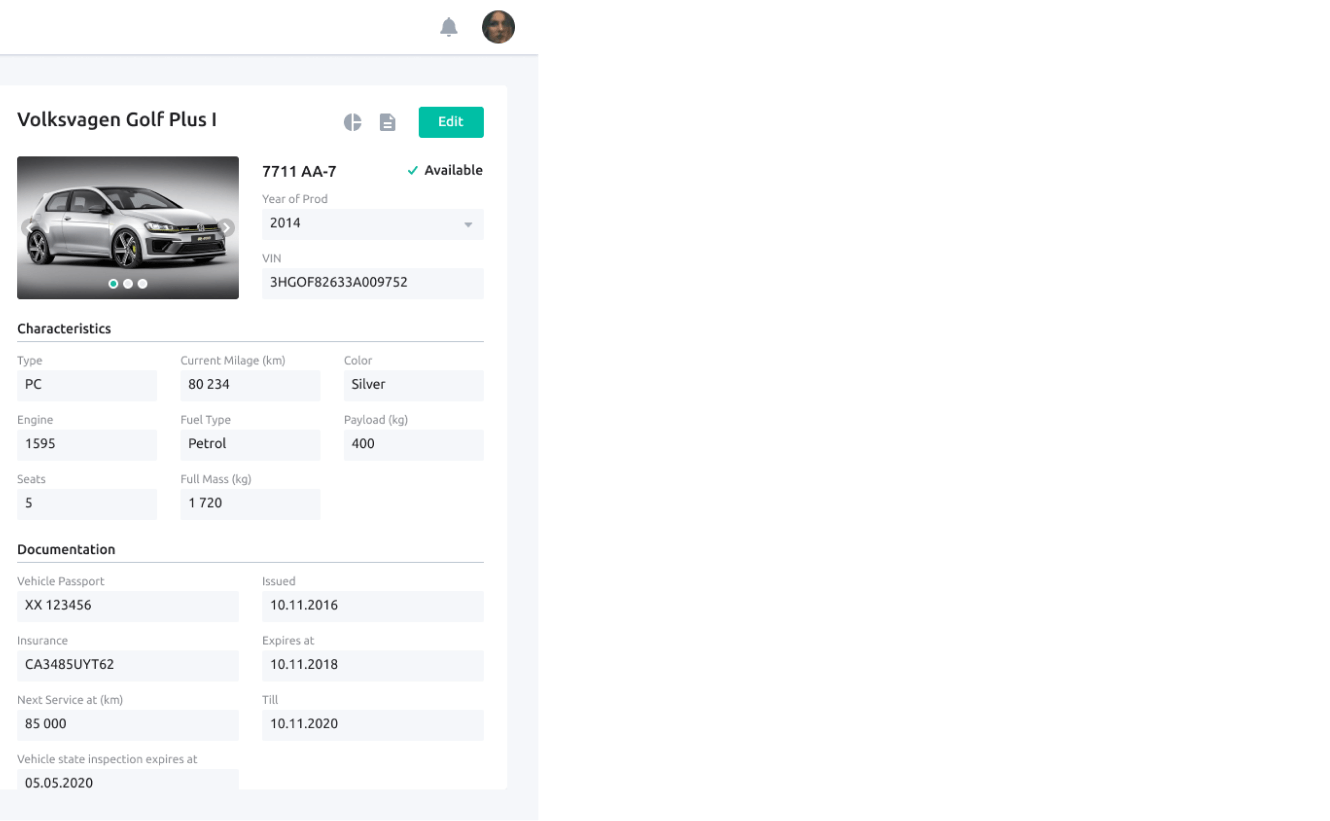This image captures a detailed section of a web page displaying information about a Volkswagen Golf Plus One. Central to the image is a rectangle containing a photo of the vehicle, which is a grayish-white color. Below the photo are three dots, the first one highlighted in green, indicating it is the selected image.

To the right of the image, there's an item number listed as 7711A8-7, signifying its catalog or reference number. The availability status is shown with both a green check mark and the word "Available." Above this status, a green "Edit" button is prominently displayed.

Further below, the web page provides in-depth details about the vehicle, including the year of production (2014) and the VIN number. A section titled "Characteristics" features multiple light gray horizontal rectangles, each containing bolded black text detailing various attributes. For instance, the vehicle type is labeled as "PC," the engine size is "1595," and the color is specified as "Silver." Other details include the full fuel type, full mass, and a payload capacity of 400.

Another section titled "Documentation" follows, containing more light gray rectangles filled with relevant information. One of these boxes specifies the next service due at 85,000 kilometers, with "85,000" prominently bolded in black text.

The entire layout is set against a clean, white background, enhancing the readability and organization of the information displayed.